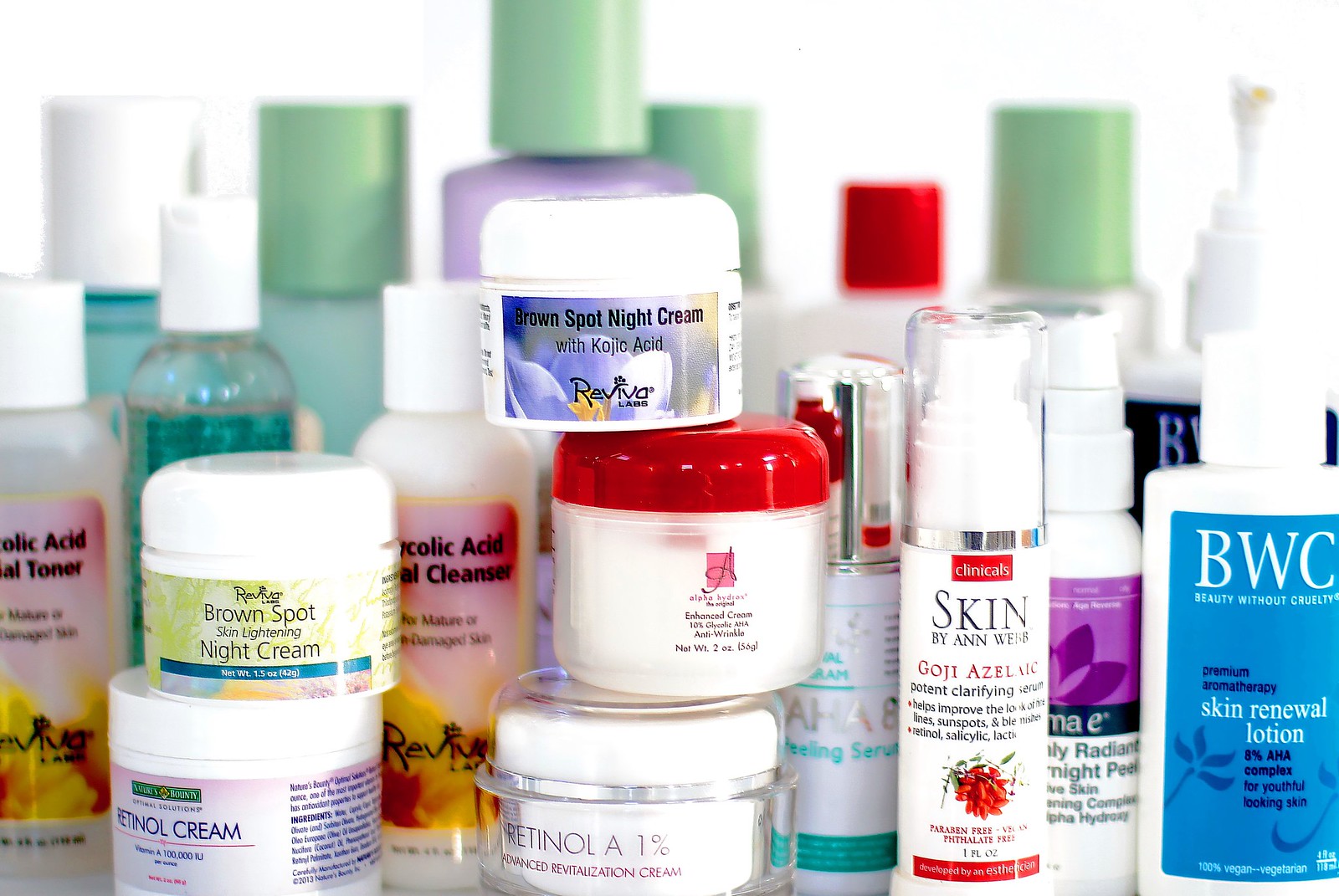This photograph showcases a diverse collection of cosmetic items neatly arranged against a plain backdrop. From left to right, the image features:

1. A small, round, yellow and white container labeled "Brown Spot Skin Lightening Night Cream."
2. Below the first container, a white and pink container labeled "Retinol Cream."
3. Adjacent to the retinol cream, a plastic bottle with a pink label titled "Glycolic Acid Cleanser."
4. Positioned next to the glycolic acid cleanser, a stack of three small cream containers:
   * The top container is white and purple, labeled "Brown Spot Night Cream."
   * The middle container, in red and white, reads "Enhanced Cream."
   * The bottom container is entirely white and is marked "Revitalization Cream."
5. Further to the right, a white and red bottle with a pump top and clear cap, labeled "Clarifying Serum."
6. Finally, a blue and white bottle labeled "Skin Renewal Lotion."

The arrangement and clear labeling of these products allow for easy identification and convey a sense of organized skincare routine essentials.